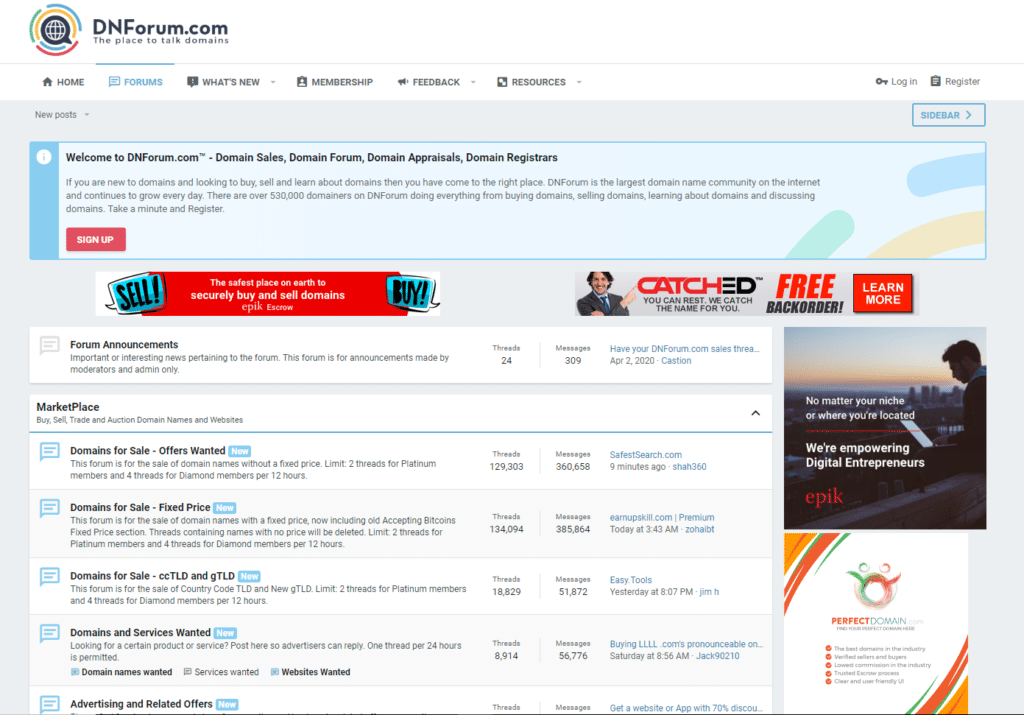Here is a detailed and cleaned-up caption for the described image:

---

The image is a screen capture from the website DNForum.com, prominently displaying the text in bold letters: "DNForum" with the initials 'D', 'N', and 'F' highlighted. The header reads, "The Place to Talk Domains," establishing the site as a specialized platform for discussions and transactions related to domain names. Below the heading, a description follows: "What is DNForum.com?" outlining the site's primary functions which include domain sales, forum discussions, domain appraisals, and domain registration resources.

Screenshot sections reveal the structured forum layout, detailing categories such as "Marketplace," where users can buy, sell, and trade domain names. Specific subsections include "Forums Announcements," "Domains for Sale - Offers Wanted," and "Domains for Sale - Fixed Price," among others. The text mentions various domain types available for transaction, like ccTLD (country code top-level domains) and gTLD (generic top-level domains), although some parts are too small to be precisely readable. DNForum.com appears to be a comprehensive resource for anyone looking to start a website or manage domain name-related activities.